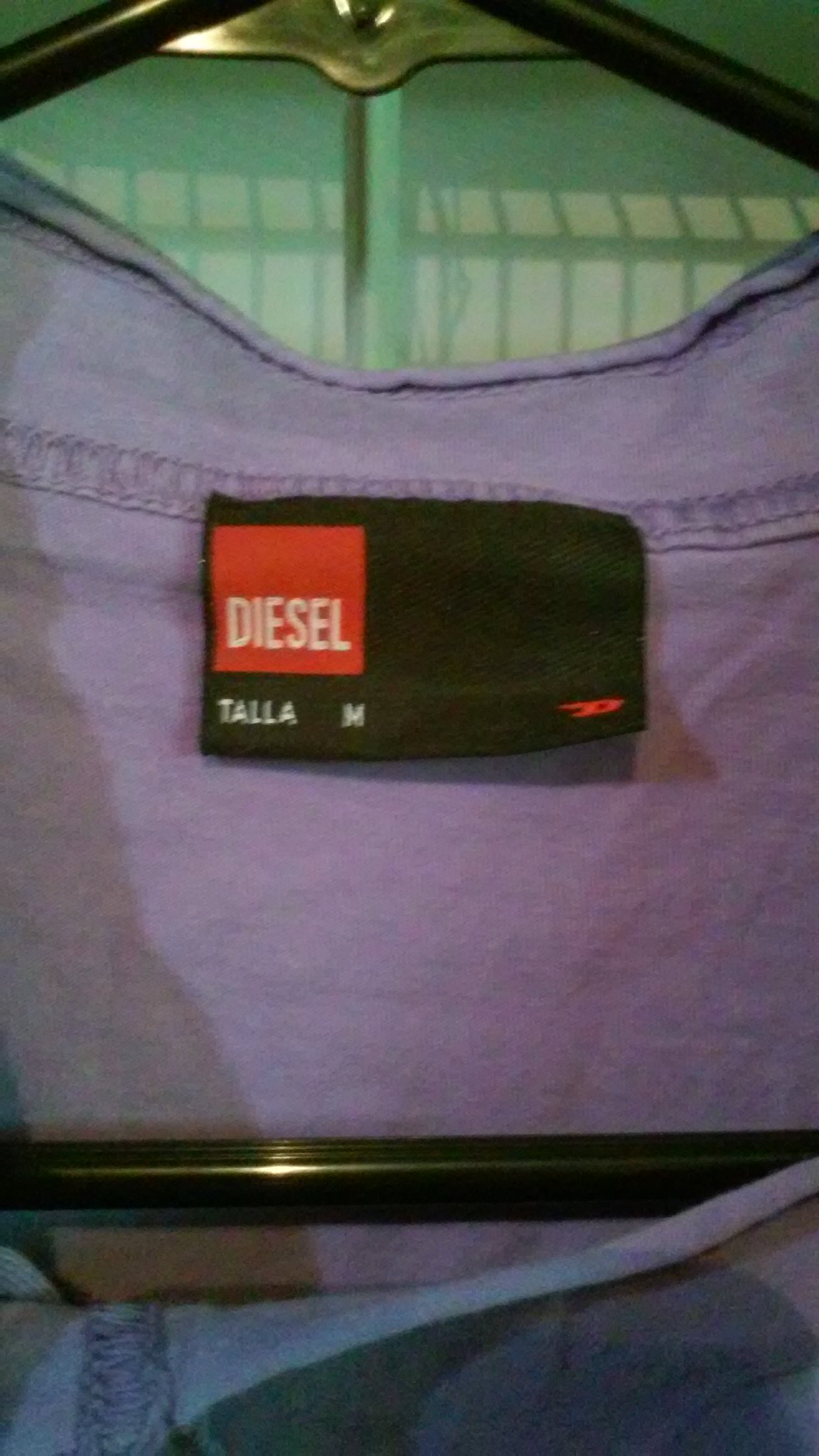The image showcases a fabric carrier or container, distinguished by a prominent rectangular badge. This badge is predominantly purple and features a smaller rectangle in the upper left corner. The smaller rectangle contains white text displaying the brand name "Diesel" and the size designation "Medium," albeit in a foreign language. Toward the bottom part of the image, a black railing traverses horizontally. Additionally, there is a brass element resembling wings, with a metal rod extending upwards to form a square frame behind it.